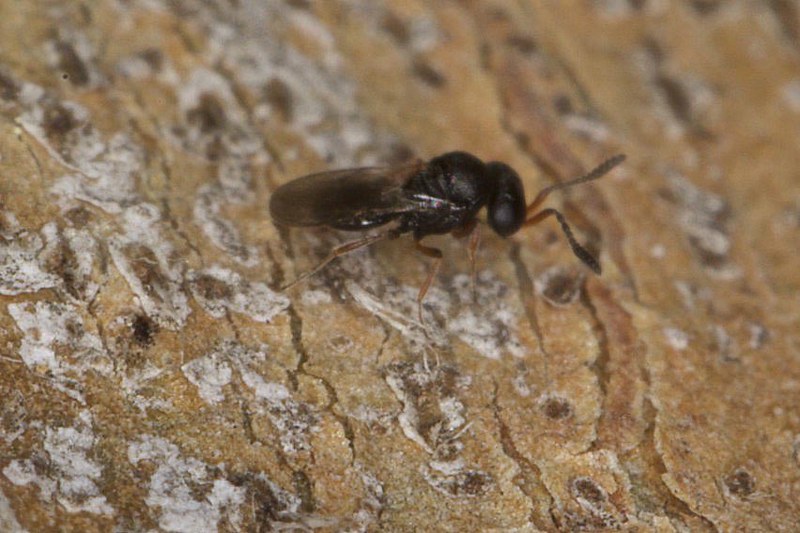The photograph showcases an extreme close-up of an insect situated on the textured surface of tree bark. The bark is light in color, peppered with small gray patches, white scales, and dark brown spots, with visible cracks and bumps. The insect, which does not resemble a bee, fly, ant, or moth, is characterized by its segmented body comprising an oblong head, a rounded torso, and an oval-shaped rear. It sports two large, orange antennae at the front of its head and has six typically insect-like hairy legs, which are also orange. The insect's body is primarily black, as are its semi-transparent wings that are tucked above its rear. The insect faces towards the right, with its head angled downward.